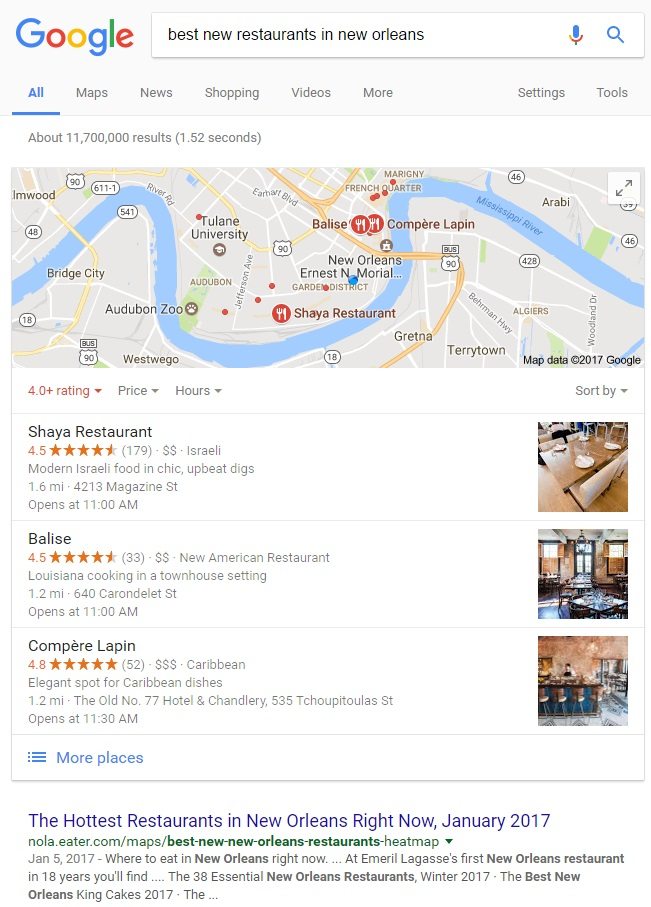This image captures a detailed view of a Google search results page for the query "best new restaurants in New Orleans." At the top of the page, a light grey background features the iconic Google logo with letters in blue, red, yellow, blue, green, and red. Below the logo, the search bar displays the query, accompanied by a microphone icon and a magnifying glass icon.

Following the search bar, a navigation bar offers options such as "All," "Maps," "News," "Shopping," "Videos," "More," "Settings," and "Tools." The "All" option is highlighted in blue, with a blue underline. The page states there are about 11,700,000 results found in 1.52 seconds, with the time indicated within parentheses.

Further down, the results feature an interactive map showing key landmarks, restaurants, cities, streets, and a river in New Orleans. Filtration options include dropdown menus for ratings (4.0+), price, hours, and additional sorting criteria.

The search results highlight three top restaurants:

1. **Shaya**:
   - Rating: 4.5 out of 5 stars
   - Reviews: 179
   - Cuisine: Israeli, Modern Israeli
   - Description: Chic, offbeat dining experience
   - Visual: Image of the restaurant

2. **Balise**:
   - Rating: 4.5 out of 5 stars
   - Reviews: 33
   - Cuisine: New American, Louisiana cooking
   - Description: Housed in a townhouse setting

3. **Compère Lapin**:
   - Rating: 4.8 out of 5 stars
   - Reviews: 52
   - Cuisine: Caribbean
   - Description: A popular venue for Caribbean dishes